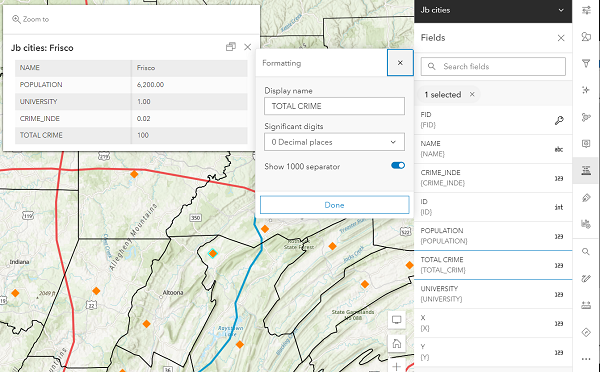A screenshot illustrates a digital map interface, though the specific location remains unidentified. Overlaid on the map are three distinct white panels. The first panel, positioned on the left, is labeled "JB Cities Frisco" and displays the population statistics for the area known as Frisco. Adjacent to it, another panel bears the title "Total Crime," formatted to display significant digits with zero decimal places. The third and larger panel to the right features an extensive menu, indicating various data fields available for research on this map: JB Cities, fields such as vid, name, crime, ID, population, total crime, and university. The setup suggests the interface is designed for configuring and analyzing geographic and demographic data.